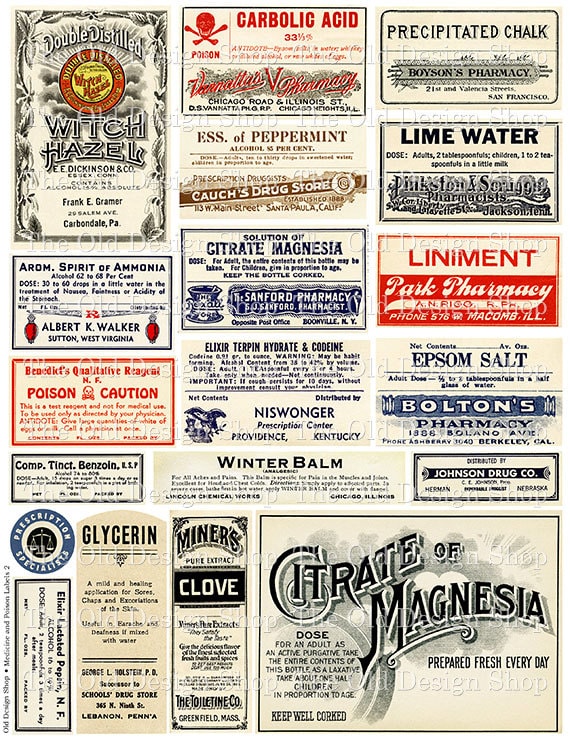The image depicts a vintage newspaper page filled with numerous rectangular advertisements for various medical and chemical items, which vividly evoke a bygone era with their distinctly 19th-century design and dual-tone color schemes. The paper itself has a yellow-tinted antiquated look, and the ads feature both bold colors like black and red, as well as simpler monochrome prints. Key advertisements include Witch Hazel in striking black and red at the top left, followed by Carbolic Acid, Precipitated Chalk, Essence of Peppermint, Lime Water with dosage instructions for adults and children, Arm Spirit of Ammonia, Citrate of Magnesia, Liniment, and several pharmacy labels such as Park Pharmacy and Johnson Drug Co. The range of products advertised spans from everyday items like Epsom Salt and Glycerine to more obscure chemicals like Benzola and Benedict's Qualitative Reagent. Each ad reflects the vintage style of that period, highlighting an eclectic assortment of pharmaceutical offerings and remedies that were once commonplace.